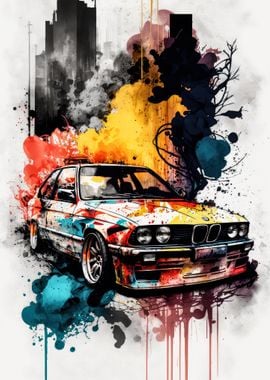The image is a small, detailed artwork of a modern coupe-like car, possibly a BMW or Mercedes-Benz, set against a white canvas background. The car is depicted using an abstract expressionist style with vibrant colors—black, yellow, red, blue, and silver—that appear to drip down the image, especially notable under the chassis. The painting is either a digitized or watercolor artwork, giving a sense of fluidity to the colors. The car is centrally positioned, facing to the right, with an elongated body and large fenders. Surrounding the car, there's an energetic mix of colors: yellow smoke and red hues billowing behind it, grey and blue splashes suggesting an urban environment, and indistinct shapes possibly representing a skyscraper and a tree in the background. The image has no identifying text or clear indicators of whether it is a photo-based digital painting or a purely hand-painted piece. The dimensions are very small, approximately an inch and a half by an inch and a half or smaller, making it a snapshot of this vivid scene.